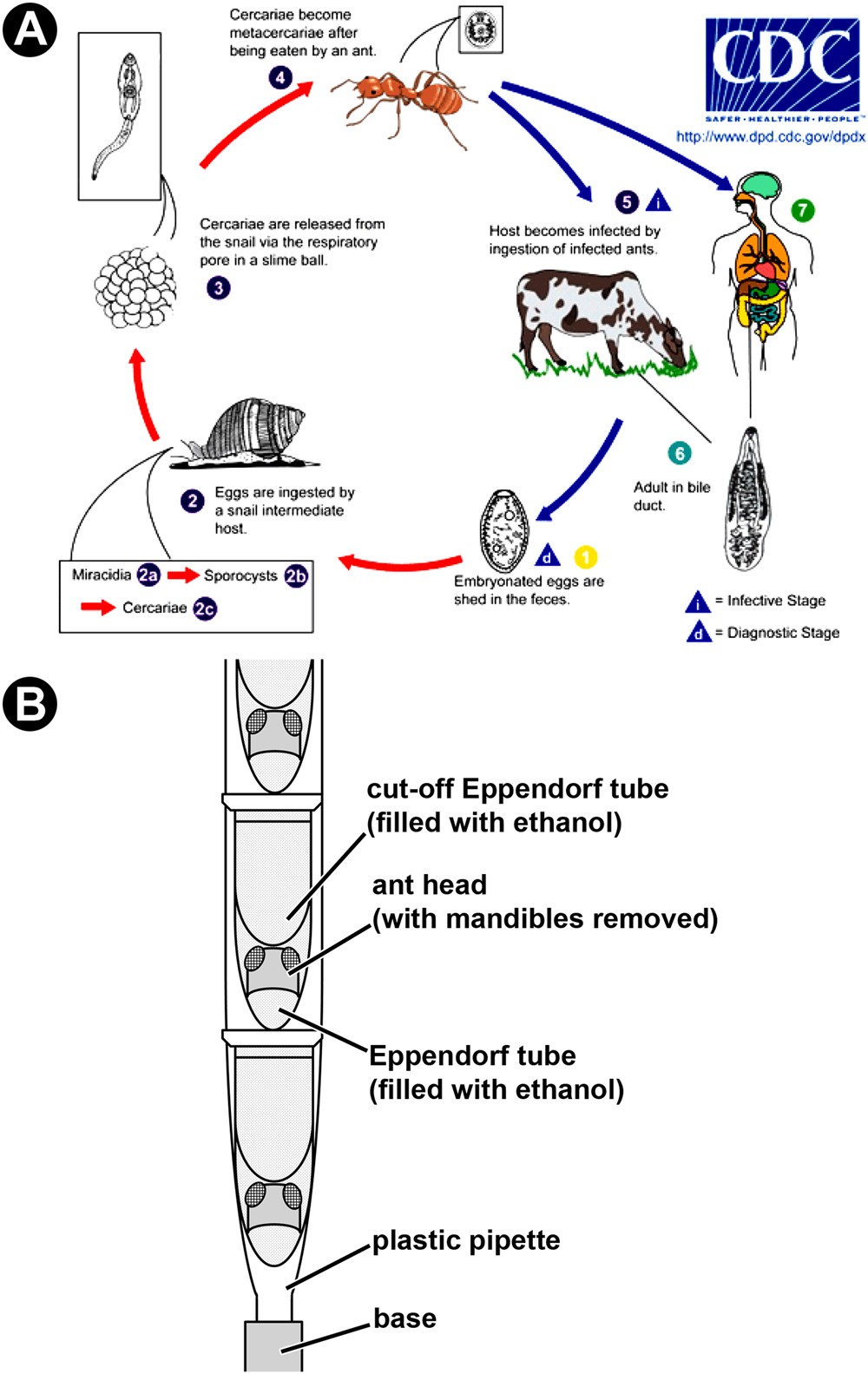The poster from the CDC features two images labeled A and B. Image A details the life cycle of an infectious organism, showcasing how embryonated eggs, shed in cow feces, are ingested by snails. These snails release larvae which are eaten by ants. These infected ants are then ingested by cows and humans, perpetuating the cycle. This part of the diagram highlights both the infective and diagnostic stages of the organism's life cycle. Image B illustrates a possible mitigation method involving a cutoff Eppendorf tube, which is comprised of a base, an ethanol-filled plastic pipette, and an ant head. This part of the diagram appears to suggest a containment or research method that could address the issues presented in A. The entire poster is branded with the CDC logo at the top right, emphasizing a focus on safer, healthier people, and references a government website for further information. The images are labeled, though quite basic in color, predominantly gray and white.